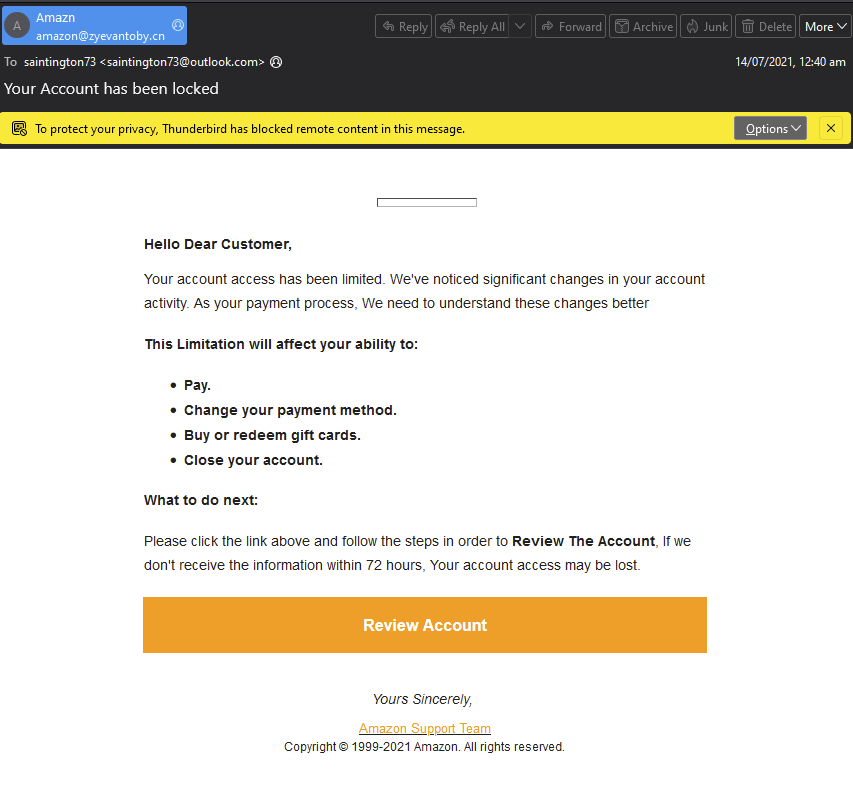Certainly! Here is a detailed, cleaned-up caption for the image description of the website:

---

The image captures a screenshot of a website with distinct sections. The top two inches of the page are black, followed by a half-inch yellow strip beneath it. This yellow section is separated from the white background, which occupies about three-quarters of the page, by a thin black border. 

In the top left corner of the black section, there's a blue rectangle featuring a gray circle on its left side containing a gray "A". To the right of the circle, the text "A-M-A-Z-N" is displayed. Below this, the text "Amazon at Z-Y-E-V-A-N-T-O-B-Y dot C-N" is visible. 

Further down, it reads "to Satington 73", followed by a greater than symbol pointing left. The text "Satington 73 at Outlook dot com" is displayed next, accompanied by another greater than symbol pointing to the right. 

Directly beneath this, bold white letters declare "Your account has been locked." The left side of the page features seven tabs that are outlined in gray and filled with black, each one labeled with text indicating different navigational options. 

Below these tabs, the date "14/07/2021" and time "1240 AM" are displayed in white text. On the right side of the yellow strip, there's a small picture icon outlined in black. Below this icon, in black text, the message reads, "To protect your privacy, Thunderbird has blocked remote content in this message."

On the right side of the screen, a gray tab labeled "Options" with white interior text and a black "X" accompanies it. 

Underneath the yellow section, a header in white text reads, "Hello Dear Customer," followed by two lines of information. Subsequently, the text indicates, "This limitation will affect your ability to," followed by a list of four potential impacts.

The page concludes with instructions on what to do next, and at the bottom, there's an orange tab approximately three inches wide, labeled "Review Account" in white text.

---